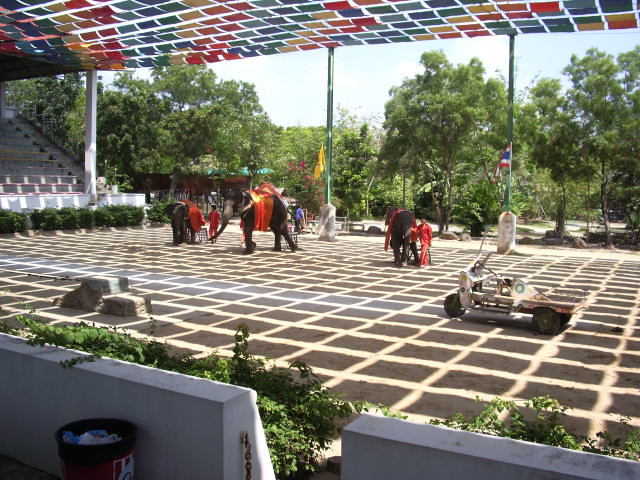On an outdoor stage surrounded by lush greenery and varying heights of trees, an array of colorful squares resembling pieces of paper on strings hangs from a roof, casting a vibrant checkerboard pattern of light and shadows onto the platform below. The sky overhead is a light blue speckled with pale white clouds, enhancing the scenic backdrop. The stage itself features several distinct elements: a white cart with three wheels, stacks of paper, and dividers made of cement blocks. In the center, three elephants adorned with red drapes stand prominently, flanked by people in red and blue attire. The people in red appear to be dressed in matching pants and tops, while one individual in a blue shirt and gray pants walks behind an elephant. Off to the left, rows of bushes mark the end of the stage, leading up to ascending bleacher-style seating. A small garbage can can be seen in the foreground, partially cut off, while a green pole-attached small vehicle rests in the bottom right corner. The top portion of the image vividly displays colorful towels or cloths in shades of red, green, blue, and purple, adding to the overall lively atmosphere.